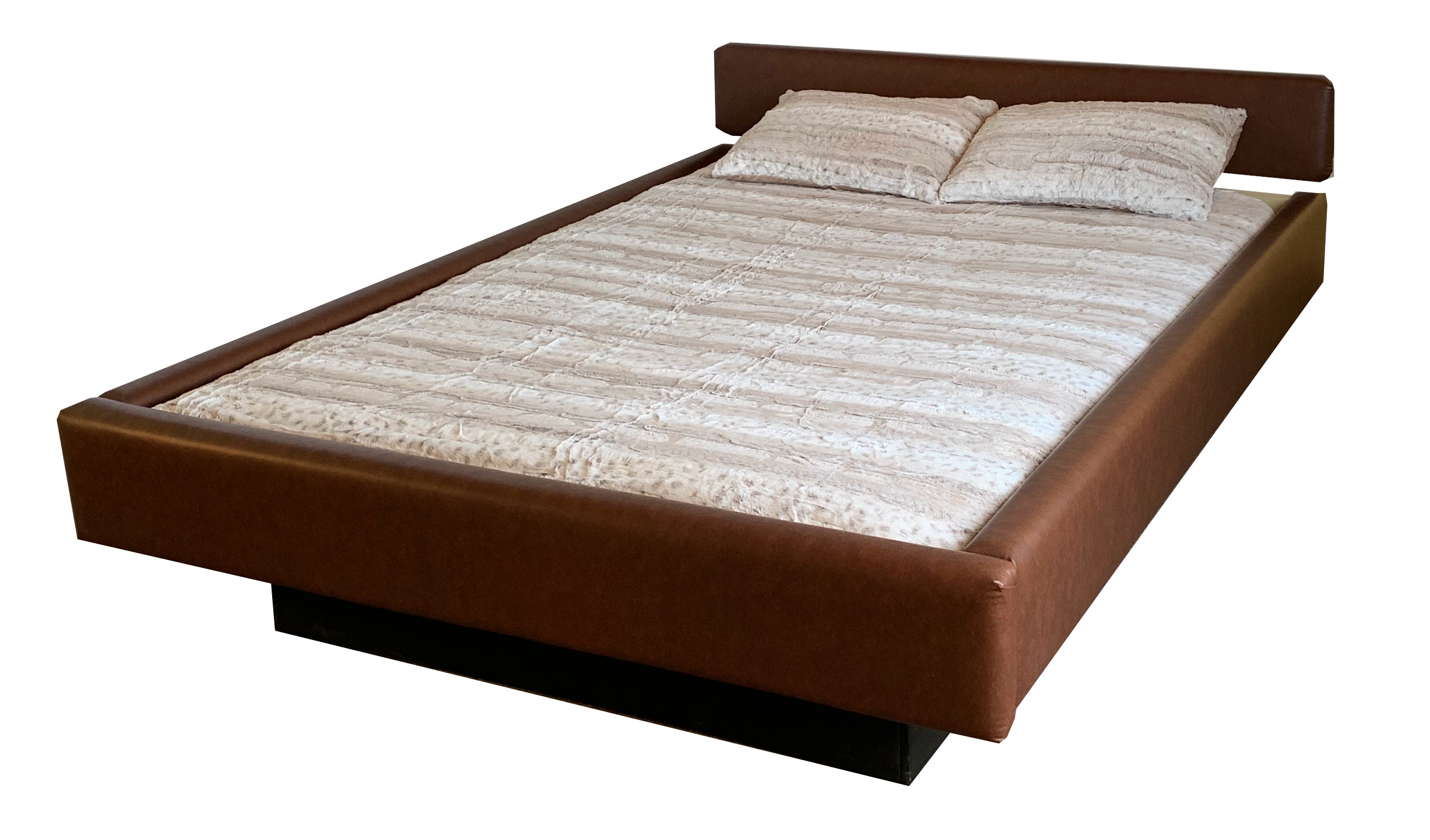The image showcases a minimalist full-size bed featuring a low-profile, brown rectangular headboard, possibly made of leather. The bed frame, outlined in brown with a black base, continues the simplistic aesthetic and remains at the same level as the mattress, contributing to its overall low and sleek appearance. The bedding consists of beige and white striped sheets, interspersed with beige dotted patterns, adding subtle texture to the design. The bed is neatly made with two pillows, each adorned with matching striped and dotted designs, positioned side by side near the headboard.